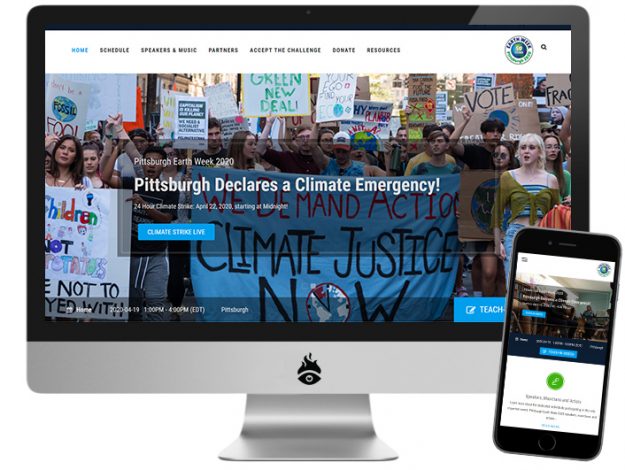This is a comprehensive description of a website dedicated to a climate change initiative. The website features prominently at the top a navigation menu with the following options: Home, Schedule, Speakers and Music, Partners, Accept the Challenge, Donate, and Resources. The homepage is highly visual, showcasing a large image of a protest, where participants are holding signs advocating for the Green New Deal and a sustainable future for children. The backdrop features a bold statement: "We Demand Climate Justice Now." 

In the foreground, significant headlines declare “Pittsburgh Declares a Climate Emergency” and highlight “Pittsburgh's Earth Week 2020” events. Another key highlight is the announcement of a "Climate Strike Live."

The website is designed to be responsive, with a mobile version that mirrors the desktop experience, ensuring ease of access on both smartphones and computers. This detailed visual and textual engagement aims to rally and inform climate activists.